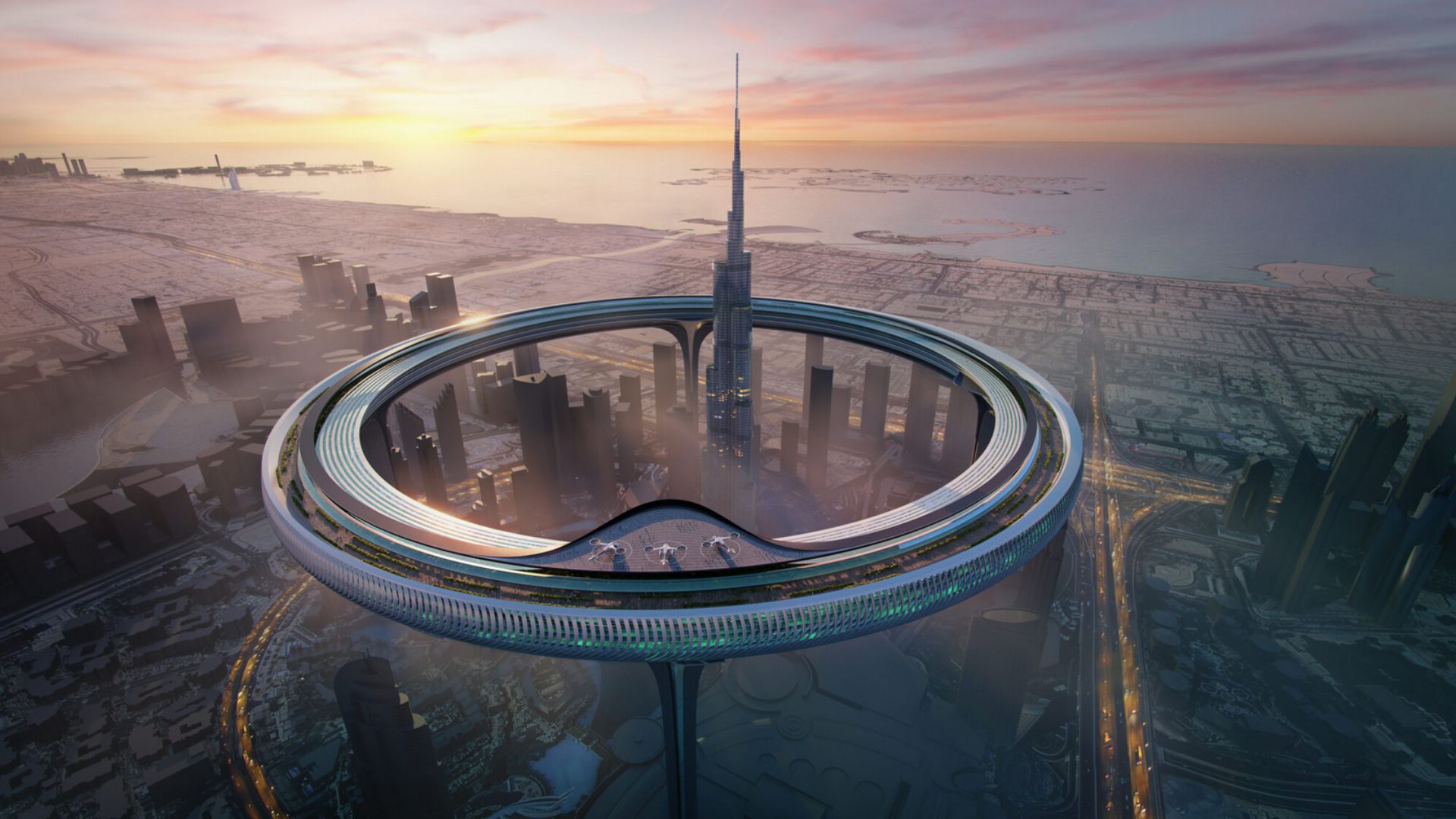The image presents a futuristic cityscape, viewed from above, positioned on the edge of a vast, grayish-blue ocean. The horizon reveals a serene sunrise, painting the sky with hues of purple, blue, and yellow, while faint yellow clouds hover around the white sunlight. The city, encased in a clear cylindrical dome, is dominated by numerous imposing skyscrapers. The tallest of these edifices boasts a spire, while others feature flat, squared-off rooftops. At the heart of this scene is a massive, futuristic hollow silver circle, perhaps a sophisticated structure or space track. This circle integrates seamlessly with the city, having a towering building with glass sides piercing through its center, accompanied by three futuristic flying crafts docked on a helipad atop one of its rings. Larger and smaller buildings spread out from this central focal point, both inside and outside the domed boundary, hinting at extensive urban sprawl. Below, roadways light up with visible traffic, and a long, sandy beachfront stretches from the left to the right, marking the transition from the urban landscape to the tranquil ocean waters.